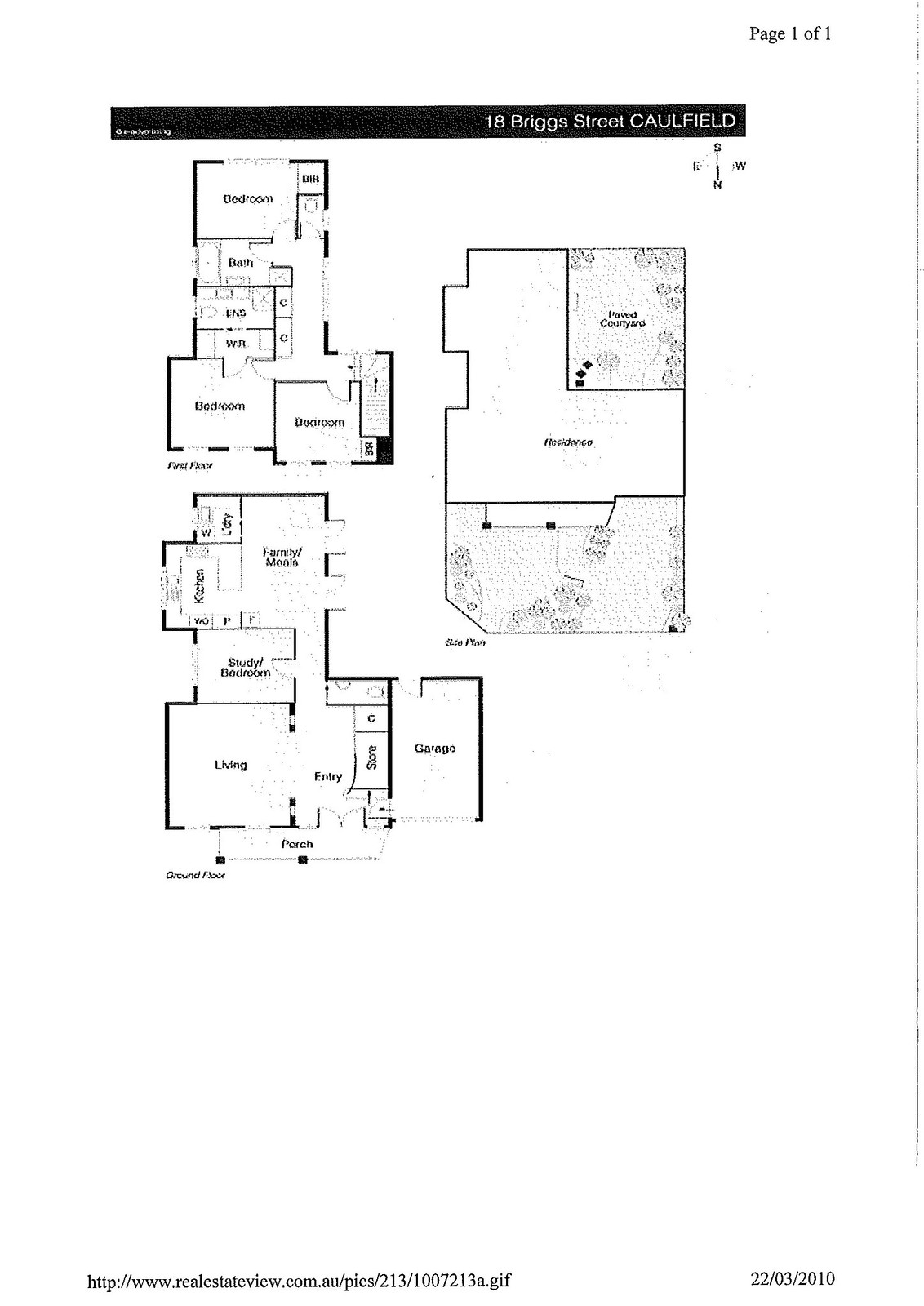Detailed blueprint of the house located at 18 Briggs Street. The first floor features a cozy bedroom and a well-appointed bathroom. Additional rooms on this level include a spacious family room and a welcoming entryway. There is also a garage providing ample space for vehicle storage and a charming porch ideal for relaxing outdoors. Upstairs, the layout includes two additional bedrooms, each designed with comfort in mind. The blueprint meticulously showcases all these elements, making it a comprehensive guide to the house's structure and design.